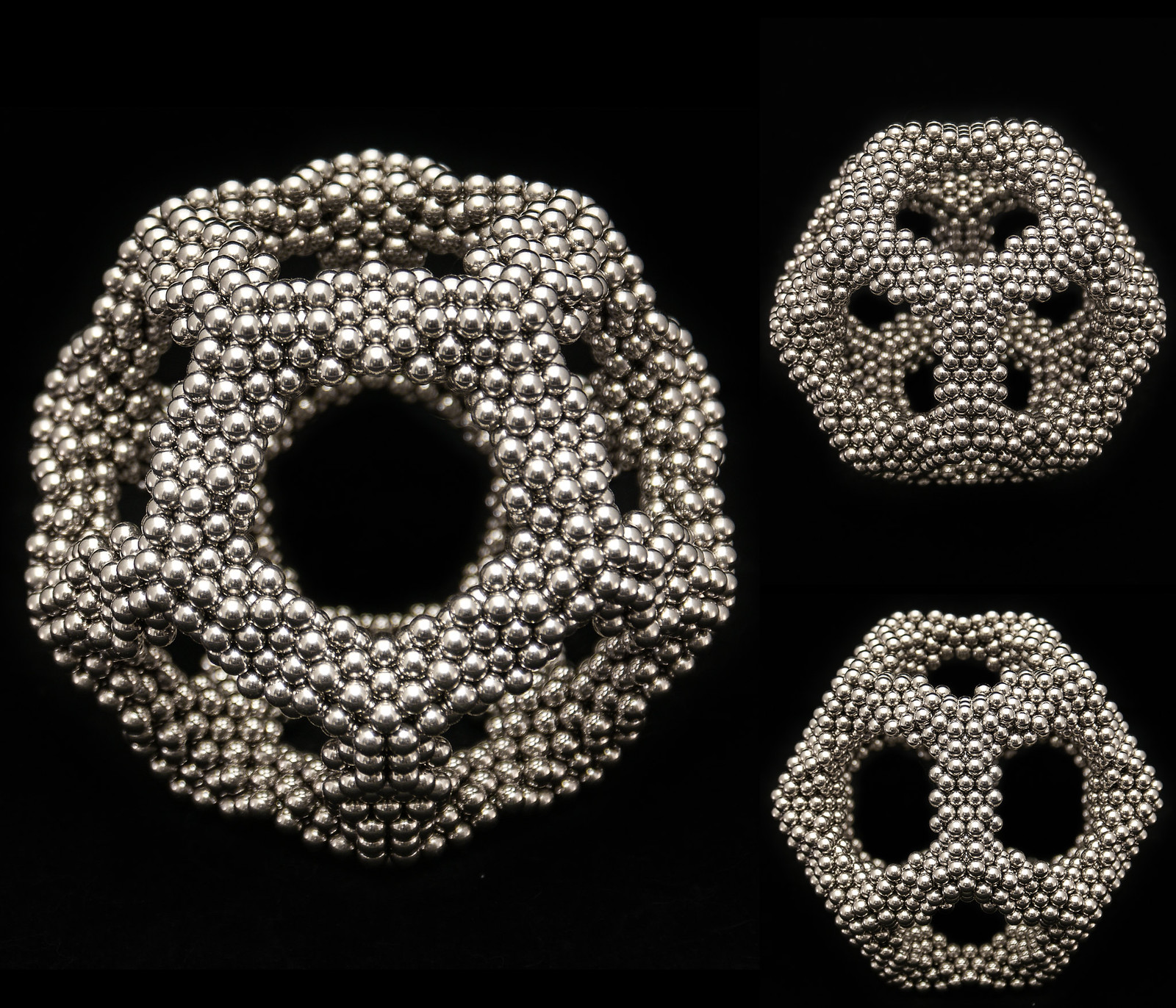The image features a sharply detailed display of three jewelry pieces set against a solid black background. On the left side, the largest piece is prominently showcased, resembling a wreath made from a multitude of small, bright, reflective silver balls. This piece has a central opening and is intricately designed, with an elevated middle section surrounded by smaller circular details. To the right, there are two smaller, round jewelry items, also composed of numerous silver beads. The top-right piece has several small openings, potentially forming a heart shape at the top, while the bottom-right piece intriguingly resembles a face, with large eyes and a small, circular mouth, complete with a hole positioned on the 'head.' Each piece is meticulously crafted, and their luminous, metallic surfaces stand out crisply against the dark backdrop.